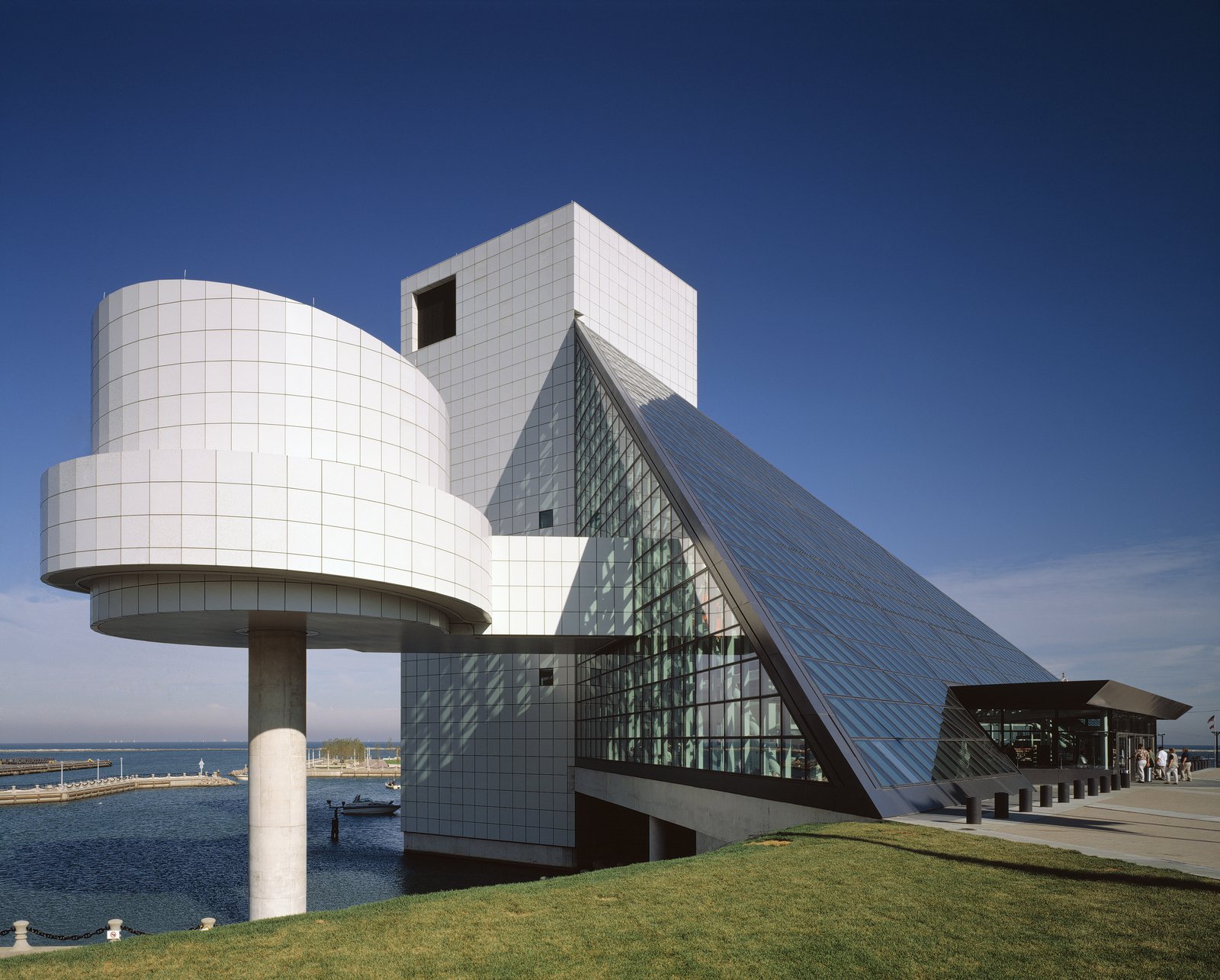In this photograph, we see a large, modern building set against a clear blue sky with hazy white clouds. The structure is primarily composed of a striking glass triangle entrance on the right side, featuring numerous square panes of glass. This leads into a tall, white rectangular building with a tiled exterior. Adjacent to the entrance is a small green grass lawn and a wide concrete slab where people are walking towards the glass doors. On the left side, there's a portion of the building extending out over a body of wavy, blue water, where a boat can be seen. A concrete pillar ascends from this area, possibly supporting a connected curvy tower. In the background, there are more clouds, a tree, piers, and distant sunlight illuminating the entire scene, suggesting a coastal location. The combination of these architectural elements and natural surroundings creates the impression of a contemporary museum or similar public space.